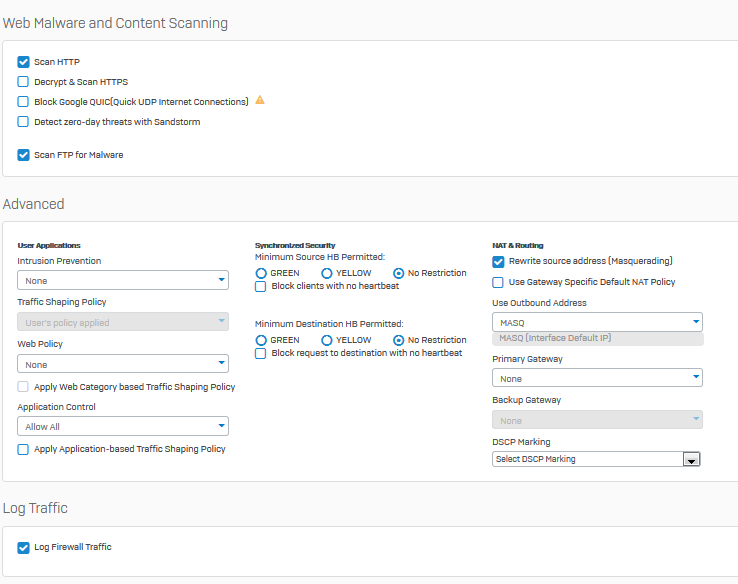This is a detailed screenshot divided into three distinct sections, each containing a white box with options and checkboxes. 

The first section, located on the left side, is labeled "Web Malware and Content Scanning." Within this section, there is a white box listing various scan options. The first checkbox labeled "Scan HTTP" is checked. In total, there are four options listed, with the last one being "Scan FTP for Malware," which is also checked.

The second section, titled "Advanced," is more complex and organized into three columns. 

- The first column is "User Applications," containing several lines of information including "Web Policy," which currently has "None" selected, and "Application Control," which has "Allow All" selected.

- The second column is "Synchronize Security." This column lists four options under "Minimum Source HP Permitted," with "No Restriction" selected for both the third and second questions.

- The third column, "NAT and Routing," features several checkboxes. The first option, "Rewrite Source Address or Masquerading," is checked, while the other options remain unchecked. Additionally, there are drop-down menus for "Primary Gateway," which is set to "None," and for "Backup Gateway," which contains some grayed-out options.

The last section is titled "Log Traffic." This section has only one checkbox, which is checked and labeled "Log Firewall Traffic."